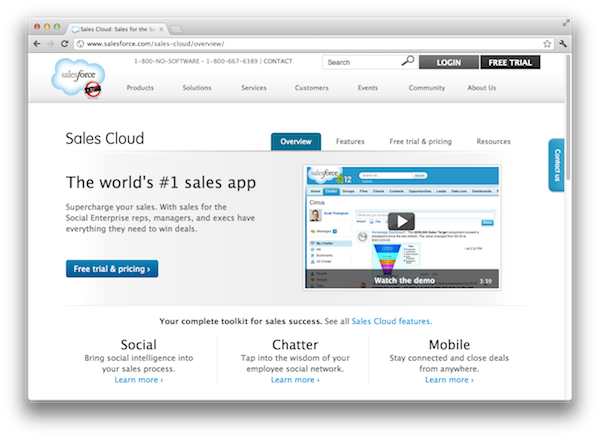Screenshot of the Salesforce App's Sales Cloud Product Page

This image captures a detailed product example screenshot of the Sales Cloud page in the Salesforce app. The top-left corner of the page prominently features the "Sales Cloud" label alongside the Salesforce icon. The regular header includes a phone number prominently displayed at the top, with a search bar positioned towards the top right. Further right, there is a login button followed by a "Free Trial" button.

Just beneath the header, a horizontal row of categories spans across the bar. The top-left section reiterates "Sales Cloud," and to its right are four additional categories: Overview, Features, Free Trial & Pricing, and Resources.

In the central section of the webpage, a noticeable video thumbnail is positioned to the right of the Salesforce page content. Adjacent to the thumbnail, bold black letters proclaim “The World’s Number One Sales App.” Below this headline is a brief description that provides more context about the app’s capabilities. Towards the bottom left of this section, a blue button labeled "Free Trial & Pricing" is easy to spot.

At the very bottom of the page, a tagline in small black letters reads “Your Complete Toolkit for Sales Success,” followed by a link prompting users to "See All Sales Cloud Features."

Continuing further down, the page is segmented into three categories: Social, Chatter, and Mobile. Each category is accompanied by a brief description and a corresponding "Learn More" button.

This comprehensive layout is crafted to provide users with an exhaustive overview and easy navigation throughout the Sales Cloud product page in the Salesforce app.